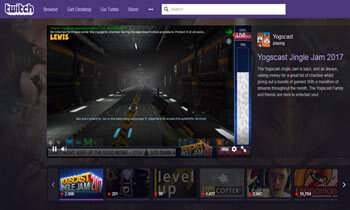In this screenshot of a web page, the top portion features a dark purple banner. In the upper left corner, there's a semi-three-dimensional logo with the text "TWITCH" in dark purple letters on a white background. The image is blurry, but it's evident that to the right of the logo, there are four areas with menu items, followed by a white search bar.

Below the banner, a screen displays content from what appears to be a video game. To the right of this screen, text reads "YOGSCAST JINGLE JAM 2017" in prominent letters. The game's visual on the screen shows a very dark hallway or possibly a subway track, adding a mysterious ambiance.

In the lower left corner, beneath the main game screen, there's a smaller, colored mini-screen. While the image quality hinders full visibility, the text “YOGSCAST” and the year “2017” are clearly written in white on a red background.